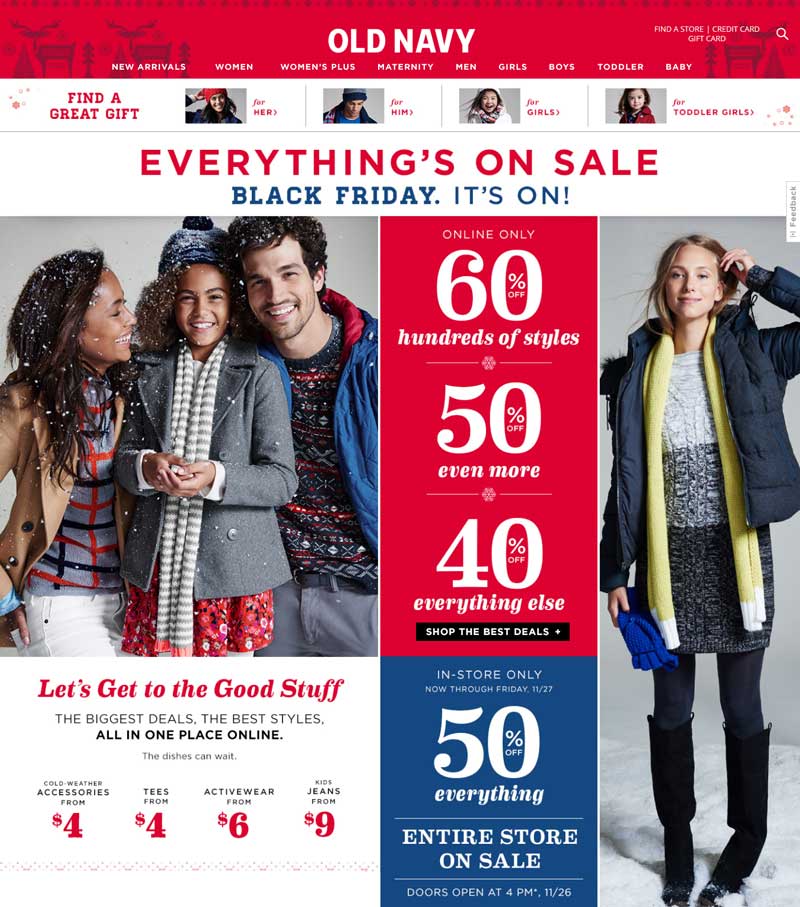The advertisement showcases a vibrant red banner across the top of the Old Navy website, featuring the brand's name in bold white font. The menu allows users to easily navigate through various categories including New Arrivals, Women, Women's Plus, Maternity, Men, Girls, Boys, Toddlers, and Babies. It also provides options to find store credit cards, and gift cards, and utilize a search bar for specific queries.

A prominent white banner underneath states "Everything's On Sale" in bold red lettering, with "Black Friday, It's On!" in smaller blue text beneath it. The advertisement emphasizes the holiday season with images of three people joyfully dressed in winter attire, with snow gently falling around them. The slogan "Let's Get to the Good Stuff: The Biggest Deals, The Best Styles All in One Place" encapsulates the excitement.

Highlighted deals include accessories starting from $4, tees from $4, activewear from $6, and jeans from as low as $9. The offer details specify an online-only discount of 60% off hundreds of styles, 50% off even more items, and 40% off everything else. In-store deals boast a 50% discount on everything in the store. The visual features a woman looking upwards in disbelief, capturing the amazement at the incredible offers.

Get ready to snag the best deals at Old Navy’s Black Friday sale!